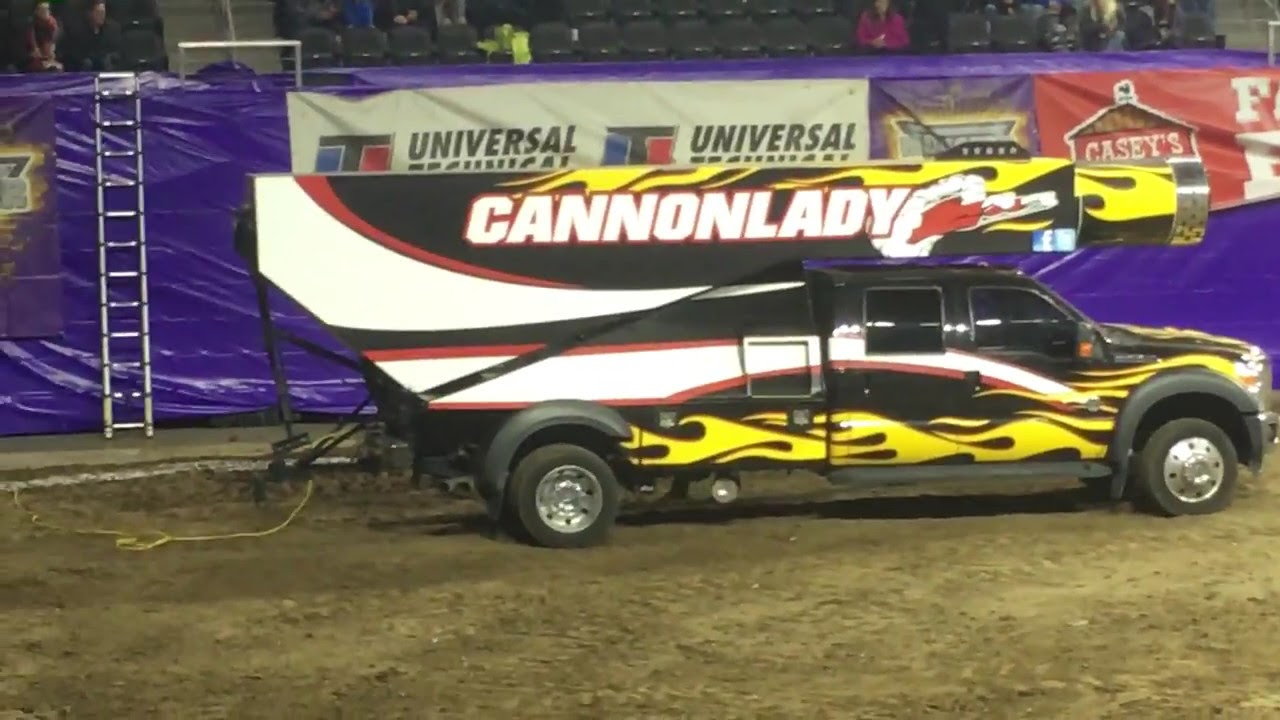In the image, there is a black truck, possibly a Ford F-150 or Dodge Ram with an extended cab, adorned with yellow flame decals and white swirls along its sides. The truck bed houses a large cannon, also featuring the flame decals and white swirls, with the phrase "Cannon Lady" emblazoned across it, accompanied by an illustration of a woman flying with smoke around her. The truck is situated in what appears to be a dirt arena, characterized by the dirt-covered ground. Behind the truck, a large purple wall or drape can be seen, featuring sponsorship banners from car manufacturers or car parts companies. Further in the background, a billboard with partially legible text advertising something related to "Universal" is visible, as well as an advertisement for "Casey's" with a barn and weather vane. The arena includes stadium seating, with several spectators visible. Additionally, a blue tarp is present, along with an extended ladder reaching up to the tarp area. The scene appears to be set up for a spectacle, possibly a car show or circus act, where the cannon may be used to shoot a performer across the arena.